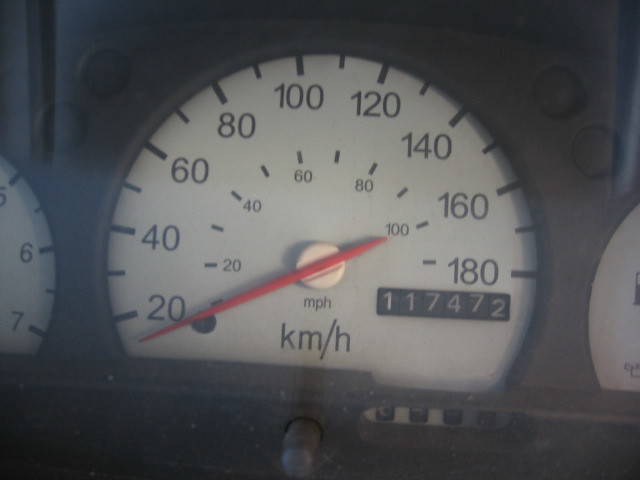This is a detailed photograph of a car speedometer, meticulously showcasing its various features. The speedometer's dial is prominently displayed, featuring black numerical markings and corresponding black dashes to denote speed increments. The numbers begin at 20, located at the 8 o'clock position, and increase in even increments (20, 40, 60, 80, 100, etc.) up to 180, which is positioned between the 3 and 4 o'clock spots. Shorter black dashes indicate intermediate speeds, such as 30, 50, 70, 90, and 110.

A distinctive red needle is centrally placed, designed to pivot and point to the vehicle's current speed as it moves. Below the dial, the text "MPH" signifies that the speed is measured in miles per hour, with a larger "KM/H" indicating the alternative measurement in kilometers per hour. Additionally, a mileage display window is situated beneath the number 180, showing an odometer reading of 117,472 miles. The design is reminiscent of classic winding dial indicators, adding a touch of nostalgia to the modern dashboard.